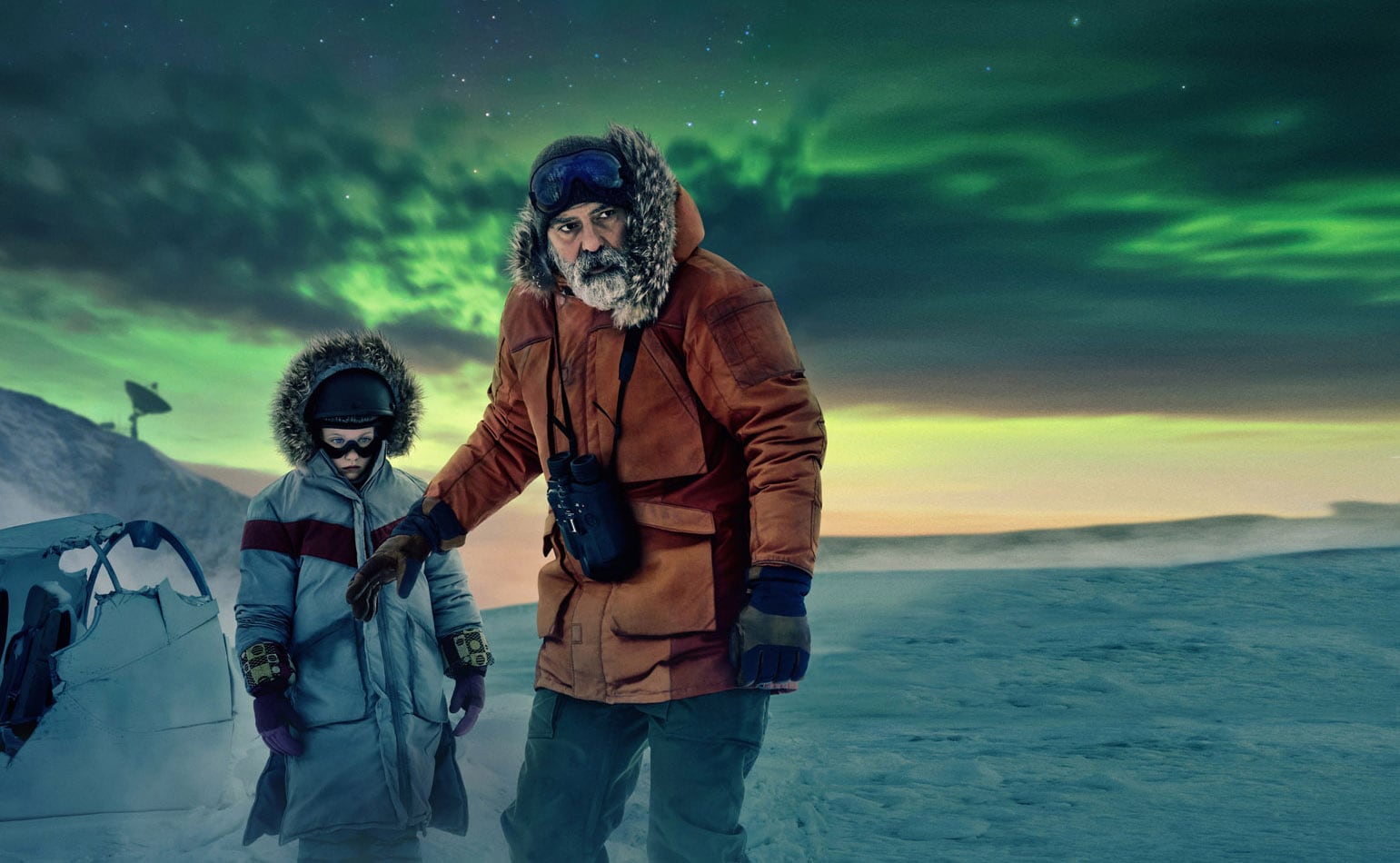In the image, an adult man and a child stand in a desolate, icy landscape, possibly the Arctic or Antarctic frontier, dressed in thick winter clothing. The adult, who bears a striking resemblance to George Clooney, wears a brown parka with a ruffed hood, a beanie, and goggles perched on his head, with binoculars hanging from his neck. The child, clad in a silver coat with a ruffed hood and blue gloves, mirrors the adult's cold-weather gear. The man extends his arm protectively in front of the child, conveying a sense of caution. Above them, the sky is adorned with a vivid aurora borealis, casting a greenish hue over the scene, while a setting sun glows faintly beneath the lights. To their left, a broken vehicle lies in disrepair, and further in the background, a satellite dish stands on the side of a hill, overlooking the flat, expansive plain with distant mountains. The overall scene suggests a moment of tension or awareness within this stark, frozen wasteland.